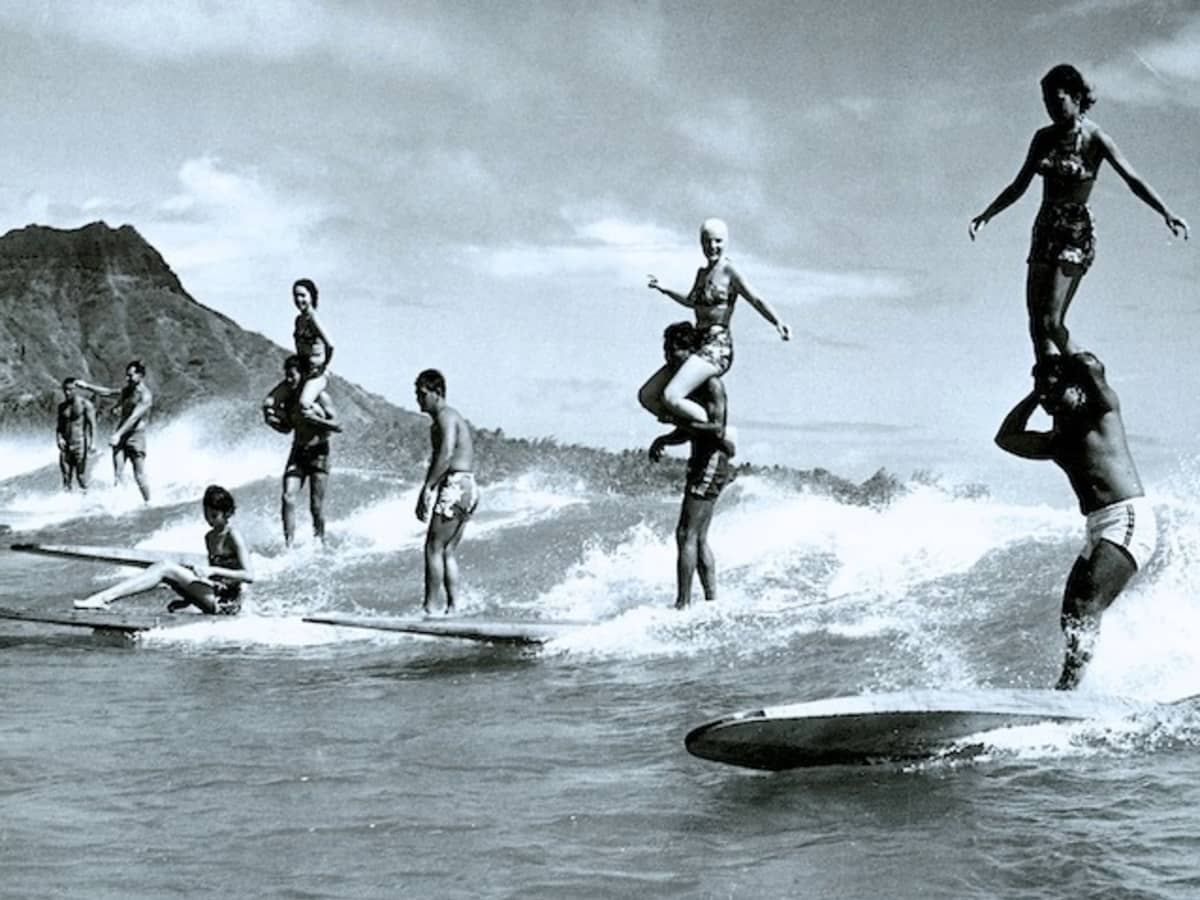This black-and-white photograph captures a nostalgic scene of surfers riding the waves in what appears to be a tropical location, possibly reminiscent of old Hawaii. Three male surfers skillfully balance women on their shoulders while riding their surfboards. The women, dressed in vintage swimwear consisting of bikini tops and shorts, add a dynamic element to the photograph. In the foreground, one man stands on his surfboard while another woman sits calmly on the front of hers. Further back, two individuals seem to be either standing in the water or on surfboards, creating a layered composition against the backdrop of a distant mound or volcanic formation. The men's swim attire includes tight-fitting shirts, adding to the overall vintage feel of this evocative image.